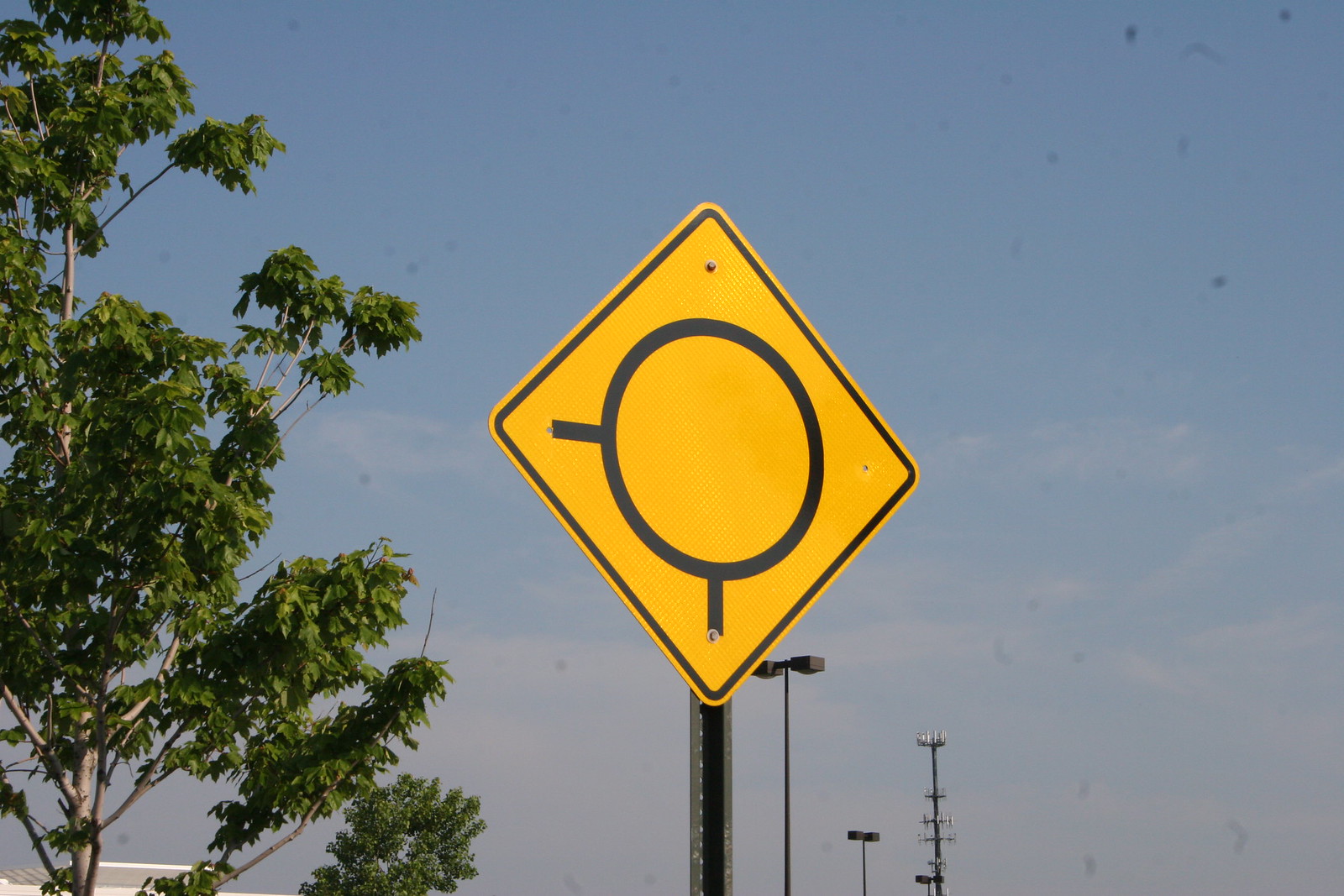The photograph captures a uniquely styled road sign, prominently placed atop a metal pole. The sign is diamond-shaped and yellow, encased in a black border, and situated against a background featuring a clear blue sky with high, wispy white clouds. A green tree is visible to the left, and the scene includes a cell tower and several parking lot lamp posts.

The icon on the sign is particularly intriguing and uncommon. At its center is a large black circle. From this circle extend two black lines: one pointing downward towards the 6 o'clock position and the other extending horizontally to about the 9 o'clock position. These lines resemble a magnifying glass with an additional attachment to the side, creating a somewhat cryptic image. The sign implies a warning or caution, possibly indicating an approaching traffic circle or roundabout.